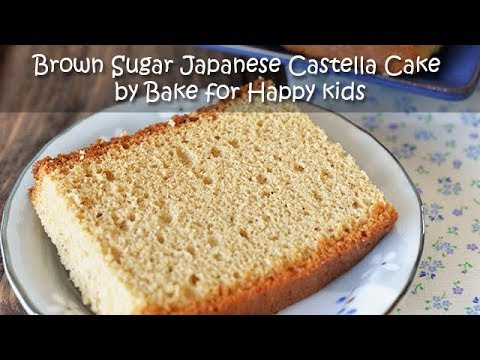The image showcases a single slice of Brown Sugar Japanese Castella Cake by Bake for Happy Kids, prominently displayed on a simple white plate adorned with a black floral border. The cake itself has a light beige, fluffy interior with darker, crisp baked edges on the top and bottom, emphasizing its spongy texture. This setup is placed on a dainty tablecloth featuring purple and blue flowers, draped over a rough brown wooden table, suggesting an informal, cozy setting. In the blurry background, a blue rectangular plate can be seen, potentially holding additional pieces of the same cake. The picture is framed by black borders on the top and bottom, enhancing its focus and giving it a polished thumbnail-like appearance. The cute, Comic Sans-style font at the top spells out the cake's name and bakery source, completing the inviting scene.